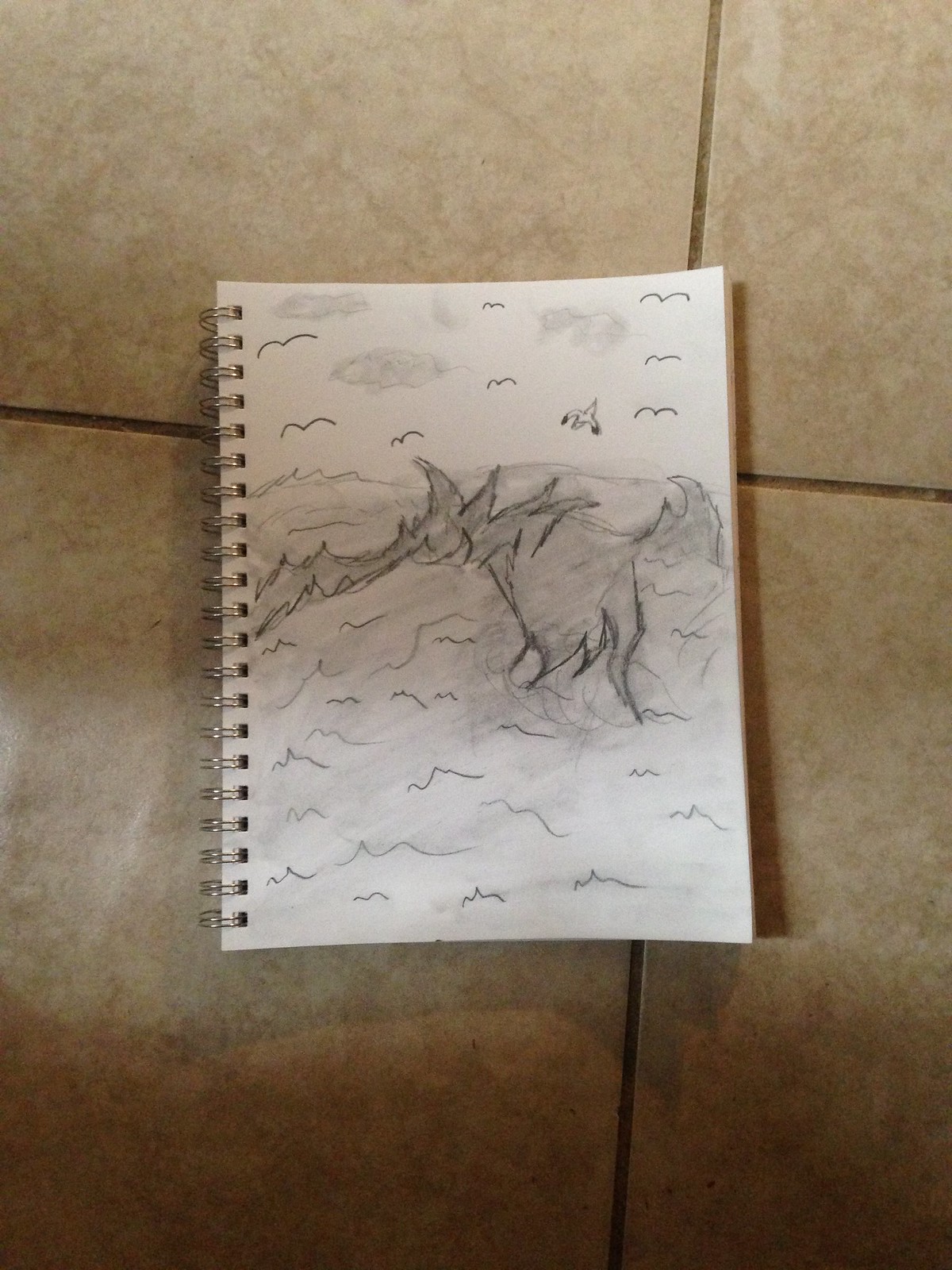This image depicts a hand-drawn artwork, created using pencil and possibly chalk, on a spiral-bound notebook placed on a marble-tiled floor. The notebook is centrally positioned in the image, providing a clear view of the surrounding large marble tiles, which appear much larger than the notebook itself, suggesting the notebook is approximately a quarter the size of a single tile. The drawing seems to be made by a child, featuring what appear to be birds represented as curved "M" shapes, along with patterns that resemble waves. The scene illustrated in the drawing is ambiguous, potentially depicting fire on the sea, though the quality of the drawing makes it difficult to interpret with certainty.